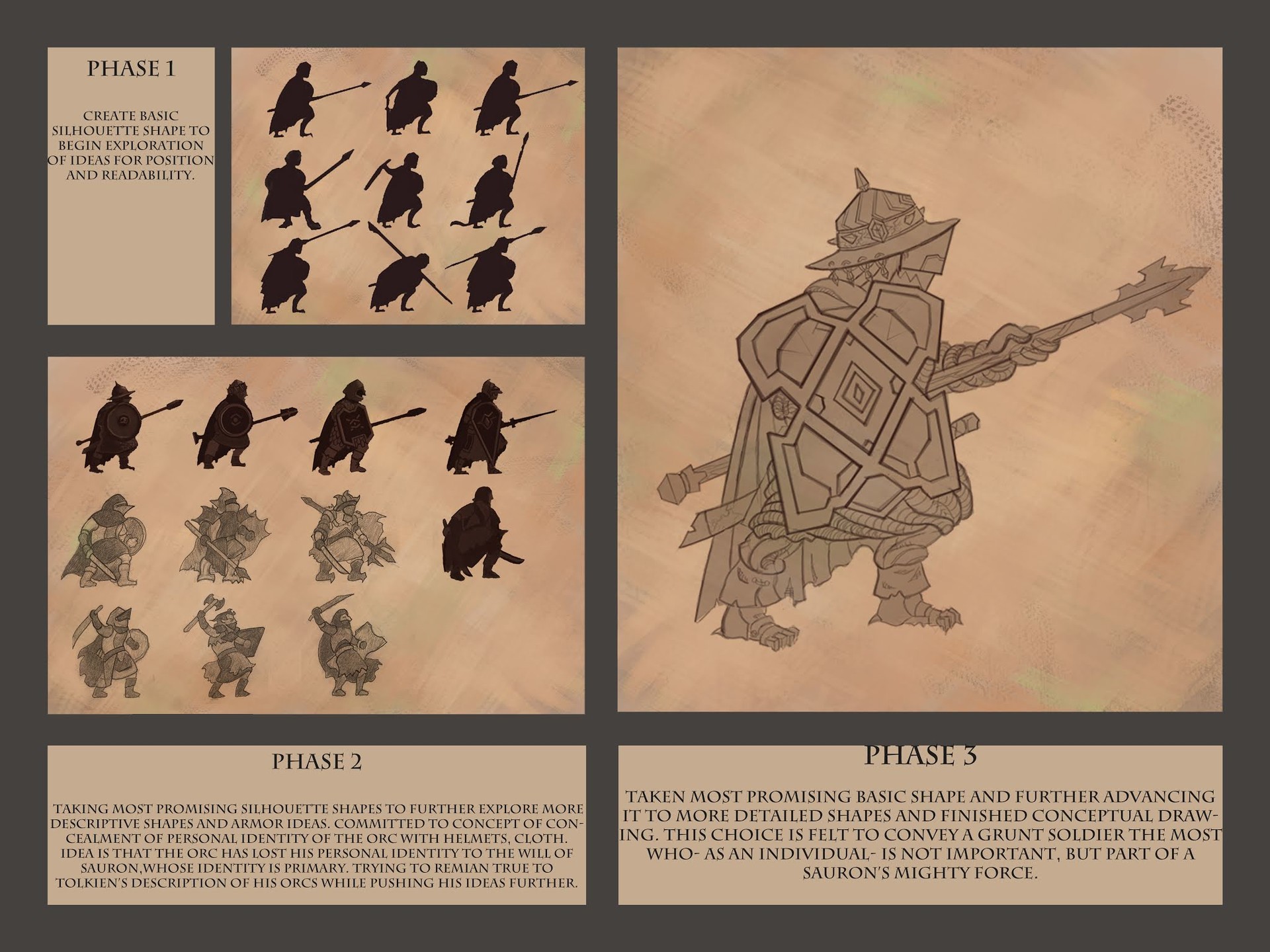The image is a rectangular diagram illustrating the design process of an orc soldier in three detailed phases. 

**Phase 1** (top left) features nine silhouetted figures of warriors holding spears and wearing capes. The accompanying text reads: "Create a basic silhouette shape to begin exploration of ideas for position and readability."

**Phase 2** (middle left) presents eleven shapes that transition from dark silhouettes to more detailed drawings of warriors with shields and spears. The text explains: "Taking the most promising silhouette shapes to further explore more descriptive shapes and armor ideas, focusing on the concept of concealing the orc's personal identity with helmets and cloth. The orc has lost its personal identity to the will of Sauron, remaining true to Tolkien's description while pushing the ideas further."

**Phase 3** (right) displays a large, detailed figure of an armored orc soldier wearing a hat, holding a spear, and carrying a shield, with its face fully covered. The text reads: "Taking the most promising basic shape and further advancing it to more detailed shapes and finished conceptual drawing. This choice conveys a grunt soldier who, as an individual, is not important but a part of Sauron's mighty force."

Each illustration highlights the progression from basic silhouettes to a fully realized warrior, emphasizing the concealment and loss of personal identity under Sauron's command.